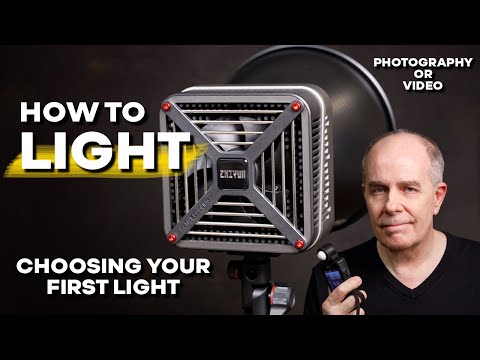This is a thumbnail image for a YouTube video with a dark background. The top right corner features white text that reads "Photography or Video." In the center, a large professional photography light, resembling a Klieg light with a silver rim and grating, displays its black outer shell. Positioned to the right of the light is an older, semi-smiling man in his 50s, with cropped grayish-brown hair and balding. He is wearing a black V-neck sweater and holding a light meter in his right hand, which is bent at the elbow. To the left of the light, white text with a yellow strip behind the word "light" reads, "How to Light," followed below by "Choosing Your First Light." The overall composition suggests the image is designed as a video cover or slide for an instructional video.